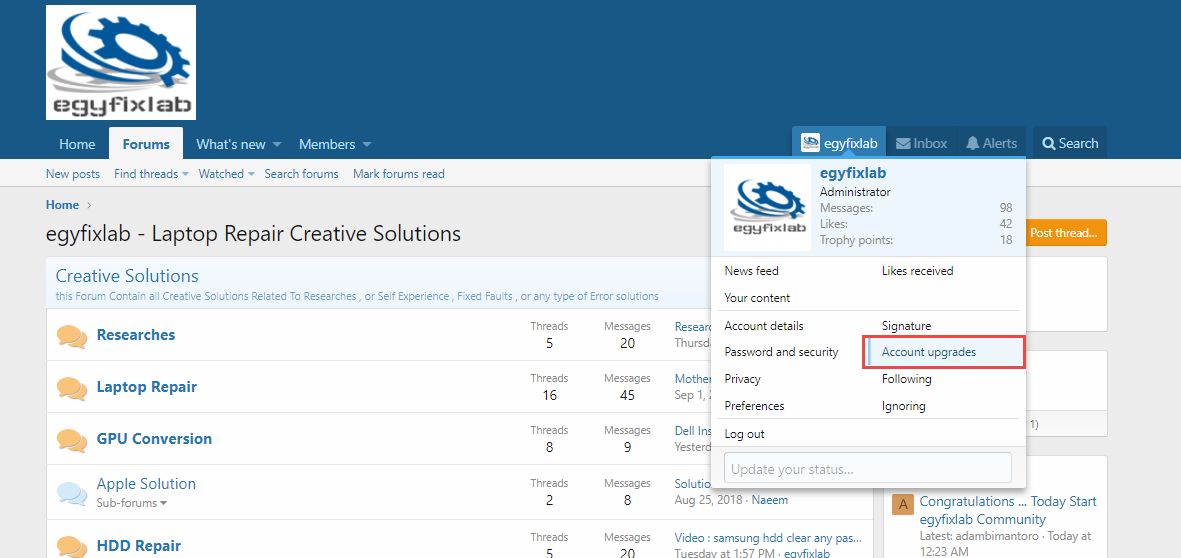This image displays a website named EggyFlexLab. The website's icon features a tool-like object surrounded by circular elements connected by a chain-like device. The main navigation bar includes several sections: Home, FEM (or possibly FUME), Forums, What's New, Members, and EggyFlexLab. Below this navigation, there are headings and descriptions for various services, such as Laptop Repair, Creative Solutions, Researchers, GPU Conversion, Apple Solutions, and HDD Repair. The site also has a section called MyFlexy. Some text appears small and difficult to read, but an "Available" status is displayed on the page.